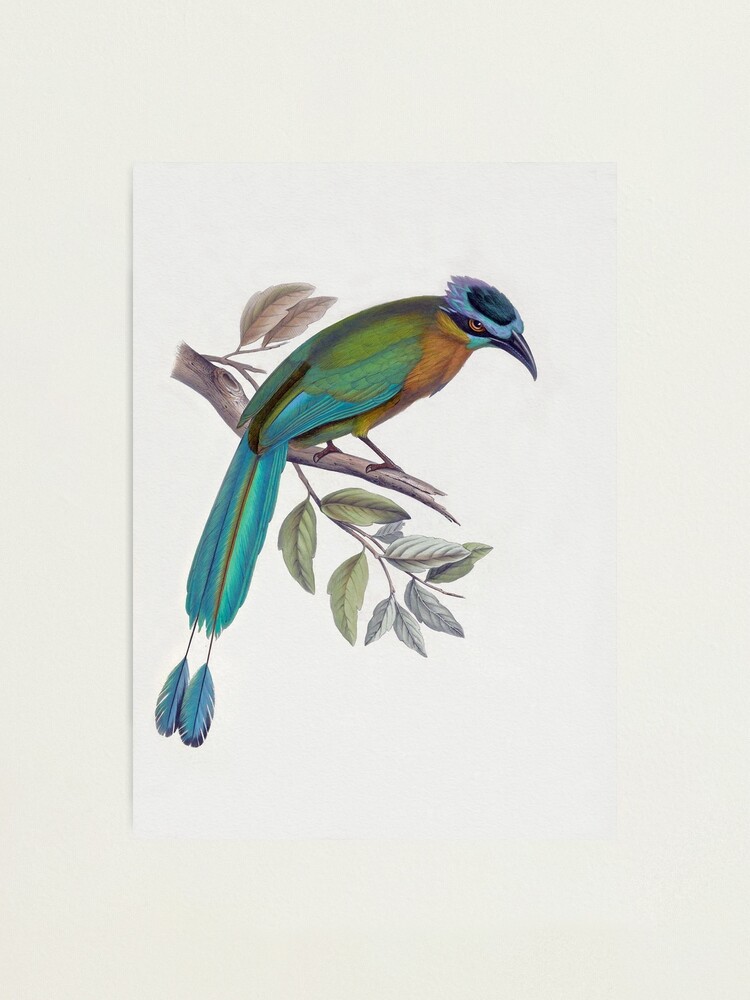This detailed illustration depicts a colorful bird perched on a light brown branch against an off-white mat background. The bird boasts a striking, multicolored plumage: its body features an orange chest, green back, and aqua-blue wings folded neatly at its sides. Its long, unique tail consists of turquoise feathers that taper into a small stem, which branches out into two smaller blue feathers. The bird's head is adorned with dark and light blue hues, with a dark brown patch at the center, giving an impression of a hat. Its eyes are a vibrant orange surrounded by a black, almond-shaped outline, adding to its striking appearance. The bird's pointed beak is dark and sharp. The branch it's perched on is accompanied by leaves in green, brown, and gray tones, adding to the natural setting. The entire scene is rendered with high detail and appears to be a finely crafted print taller in orientation than it is wide.